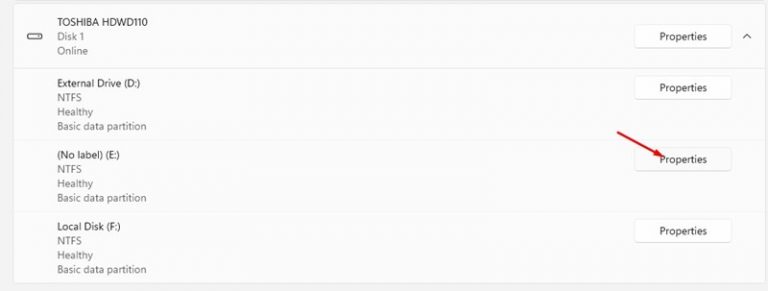The image displays a computer screen showing system information for an external hard drive and its connected devices. The interface highlights the storage details and statuses of the drives linked to the system. 

At the top is "Toshiba HDWD110 (Disk 1)," indicated as "Online." Adjacent to it, there is a "Properties" button, presumably for accessing and modifying the drive settings.

Beneath this, the display lists:
1. "External Drive (D:)," labeled as "NTFS Healthy" and categorized under "Basic Data Partition," with the "Properties" option next to it.
2. "No Label (E:)," also marked as "NTFS Healthy," classified as a "Basic Data Partition," featuring a marked "Properties" button, distinguished by a red arrow pointing to the "R" in "Properties."
3. "Local Disk (F:)," similarly described as "NTFS Healthy" under the "Basic Data Partition" category, with the "Properties" option available.

The interface uses a simplistic, monochromatic design with a black-and-white color scheme. Text is black on a white background, and each "Properties" button is encapsulated in a white box, emphasizing a straightforward, user-friendly layout.